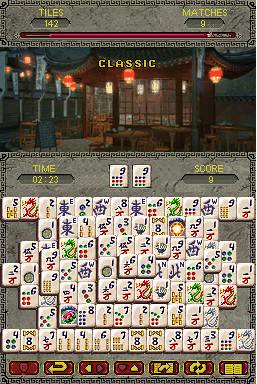This image is a screenshot from a video game, displaying a rectangular interface that is taller than it is wide. The top left corner shows "Tiles: 142," while the top right corner lists "Matches: 9." An energy bar is also visible in this area. Below this, the time reads "2 minutes and 23 seconds," and the score is listed as "9" on the right.

The top section features a detailed visual area displaying a room with a traditional Asian building resembling a pagoda, adorned with red and white lanterns. This central structure has a roof that curves upwards, flanked by windows on two sides.

Below the visual area, there are several rows of tiles, likely six or seven, arranged in different configurations. These tiles have various drawings and symbols, including dots and a dragon, with some featuring Asian characters, making up a significant portion of the screenshot. At the bottom of the screen, there are controls represented by red buttons.